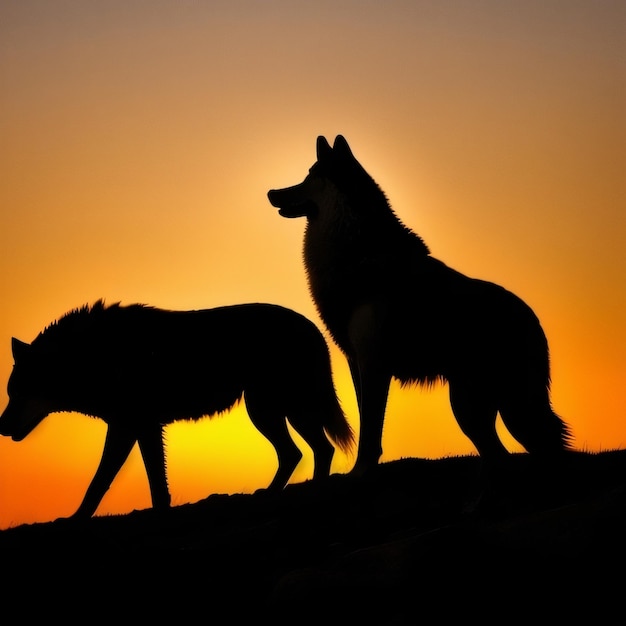This professionally done photograph captures a breathtaking post-sunset scene in nature, rendered in a vertical orientation. The sky is a mesmerizing gradient of colors, transitioning from a yellow horizon through shades of orange and pale orange to a brownish hue at the top. The ground forms a solid black silhouette with tufts of grass visible, positioned higher towards the right side.

Dominating the foreground are two striking black silhouettes of wolves, accentuated against the vivid sunset backdrop. The first wolf, located towards the left, appears to be slinking with its head lowered and mid-step, moving to the left. The second wolf, on the right, stands more upright, with its head raised, pointy ears, and a fluffy tail visible. Though only three legs are discernible, it is also stepping towards the left. The entire scene is an epitome of natural beauty and precise craftsmanship, capturing the essence of wildlife against the enchanting colors of a setting sun.